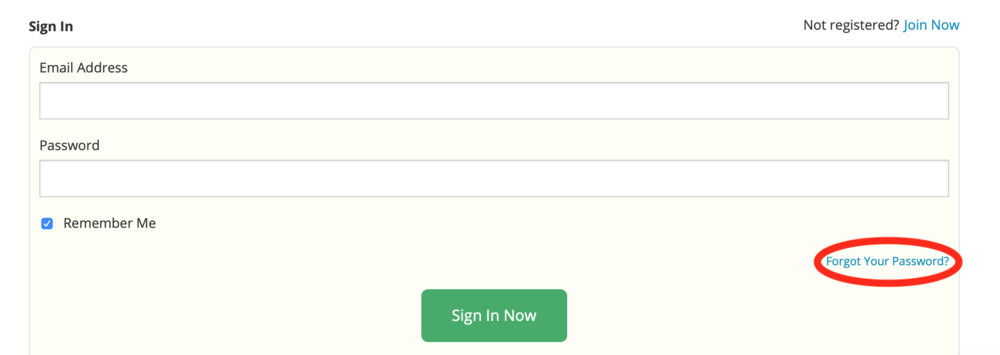The image depicts a sign-in pop-up set against a cream-colored background. On the left side, users are prompted to sign in, while the right side offers an option to join if not registered, emphasized with a blue "Join Now" link. 

In the center is a section for entering an email address, featuring a white data field. Directly below is another data field for the password. Beneath the password field, a "Remember Me" checkbox is prominently checked, highlighted in blue.

On the right side of the form, a "Forgot Your Password?" link is encircled with a thick red oval, likely added using a photo-editing tool, suggesting attention to this option. 

Centered at the bottom of the pop-up, there is a green "Sign In Now" button with white text. The overall design is minimalist, utilizing a clean palette of black, white, cream, blue, green, and red. The pop-up is horizontally elongated, indicating a landscape-oriented rectangle. The simplicity of the design suggests a focus on functionality without any additional content or context about the website.